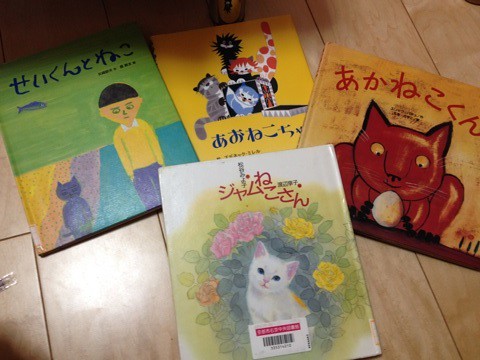This image captures a top-down view of four vibrant children's books lying on a wooden floor with wide, interconnecting slats. Each book prominently features a cat illustration on its cover and is inscribed in an Eastern script, which is not Chinese but could be Japanese or another Eastern language. 

The book in the top left corner has a colorful cover with a small blue cat standing next to a young boy sporting a dark bowl haircut, a yellow long-sleeved shirt, and blue pants. The boy appears to be outlining or doodling the cat. 

To its right, the second book with a yellow cover showcases four cartoonish cats in different colors: gray, blue, red with white polka dots, and black. 

The third book, positioned further right, displays an enormous red cat with a white paw sticking out, seemingly holding a white egg or ball in its paws against a deep yellow background with red script.

Below these three, the fourth book with a predominantly white cover features a gentle white furry kitten with pink ears sitting amidst a garden of pink, yellow, and orange flowers. This book exudes a distinct charm with its colorful floral border and has a yellowish hue around the image reinforcing its lively and cheerful theme.